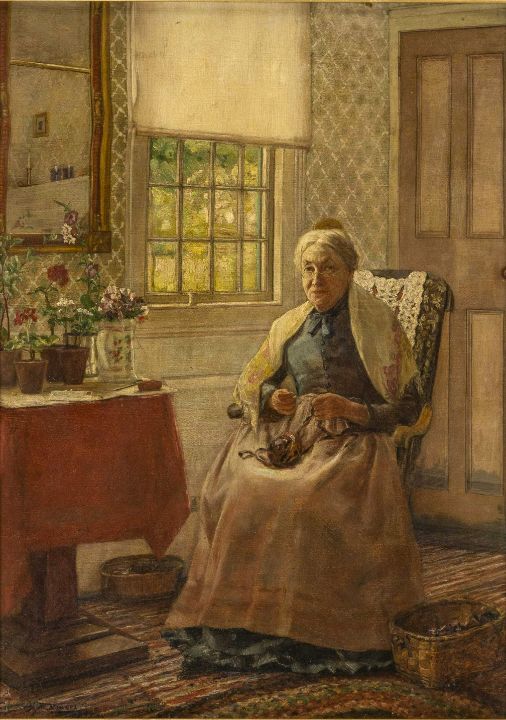This painting captures an old woman seated in a dark brown wooden rocking chair, her figure gracefully reflected in a mirror situated at the top left corner. The woman, with her gray hair meticulously balled up and secured, wears reading glasses resting on her nose. She is adorned in a long-sleeved, navy blue dress complemented by a large white apron that drapes down to her feet. A white scarf or blanket is elegantly draped over her shoulders.

Her nimble fingers work with yarn, likely preparing to knit, as small baskets containing additional yarn sit at her feet. To her left, a small table covered with a vibrant red tablecloth displays various potted plants with flowers in red, white, and purple hues. Further accentuating the scene, a window with a partially open blind allows daylight to stream into the room, revealing a glimpse of green foliage outside. Behind her, a brown wooden door stands closed, and the room's decor is completed by gray wallpaper and carpet flooring. The edges of the image are notably crisp, suggesting it could be a scan or photograph rather than a traditional painting.